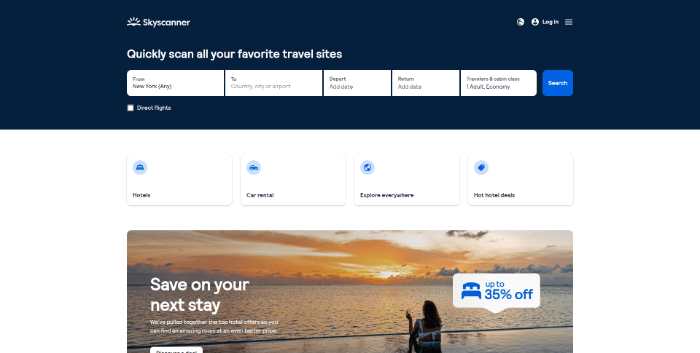In this image, we are looking at the homepage of the travel website Skyscanner. At the top of the page, the site’s name is displayed prominently in white letters. To the right, there is a login area featuring three horizontal white lines, symbolizing additional options, alongside an icon of a person indicating the user account section.

Within a dark blue rectangle that spans the search area, there's a tagline that reads, "Quickly scan all your favorite traveling sites." The search functionality allows users to enter their departure details, with fields labeled "From," "To," "Depart," and the option to add another date. Following these fields, a blue button is available to initiate the search process. There are five distinct options provided for users to customize their search.

Below the search bar, there are further options categorized under "Hotels," "Car Rental," "Explore Everywhere," and "More Hotel Deals," catering to various travel needs.

Dominating the lower section of the page, there's a captivating image of a woman seated on a beach, gazing out at the ocean during sunset. A sign on this image advertises discounts of up to 35%. Positioned on the left side of the image, a message in bold white letters invites users to "Save on your next stay."